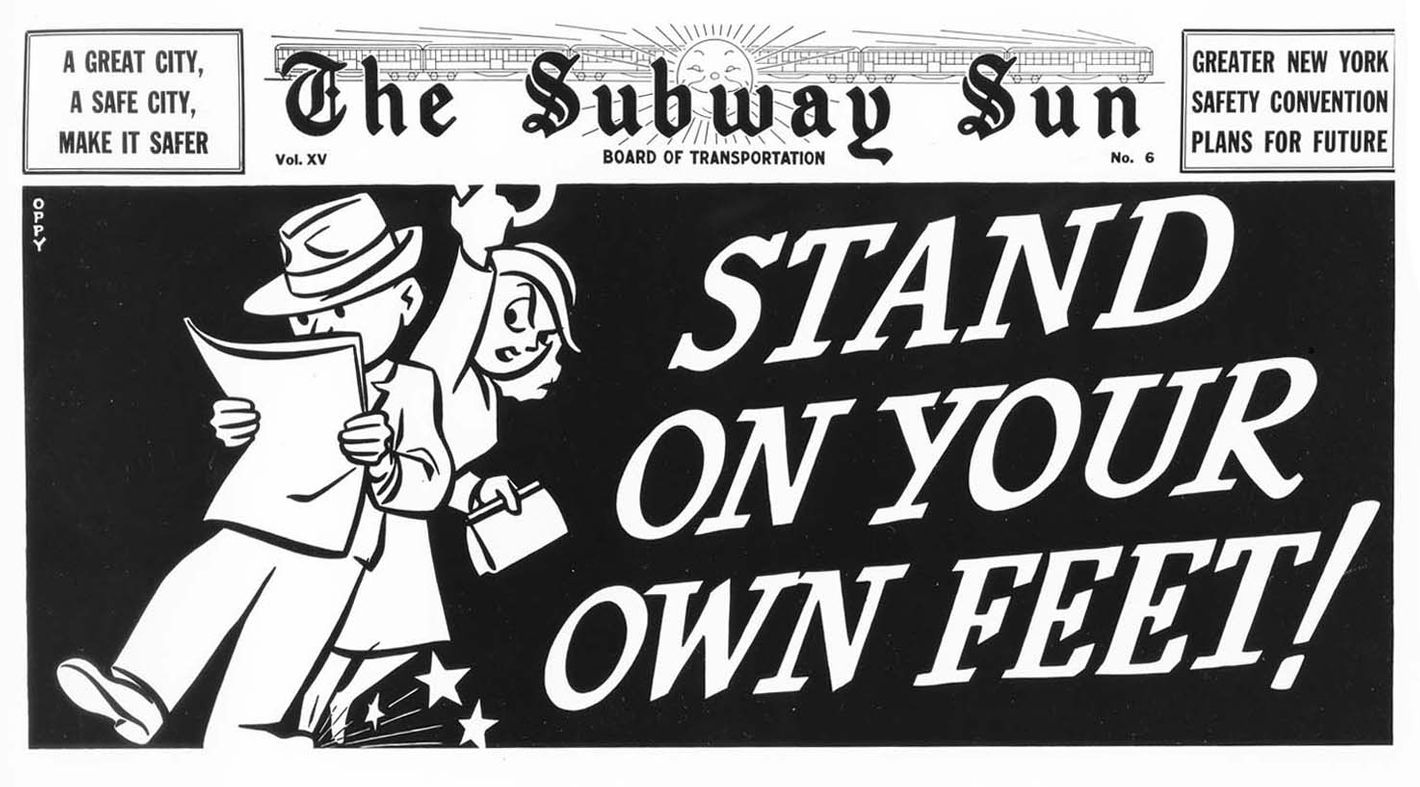The newspaper clipping, originating from "The Subway Sun" by the Board of Transportation, prominently features a safety message. In the upper left corner, within a black border text box, it declares, "A great city, a safe city, make it safer." On the upper right, the text reads, "Greater New York Safety Convention Plans for the Future." The main visual depicts a man and a woman in a comic-style illustration. The woman, dressed in a hat and clutching a train handle overhead, looks irritated as the man, also wearing a hat and leaning back, appears oblivious, engrossed in his newspaper. At the bottom, against a solid background, bold white text commands, "Stand on your own feet!" This striking design is entirely in black and white, highlighting the safety message with clear and intense contrasts.